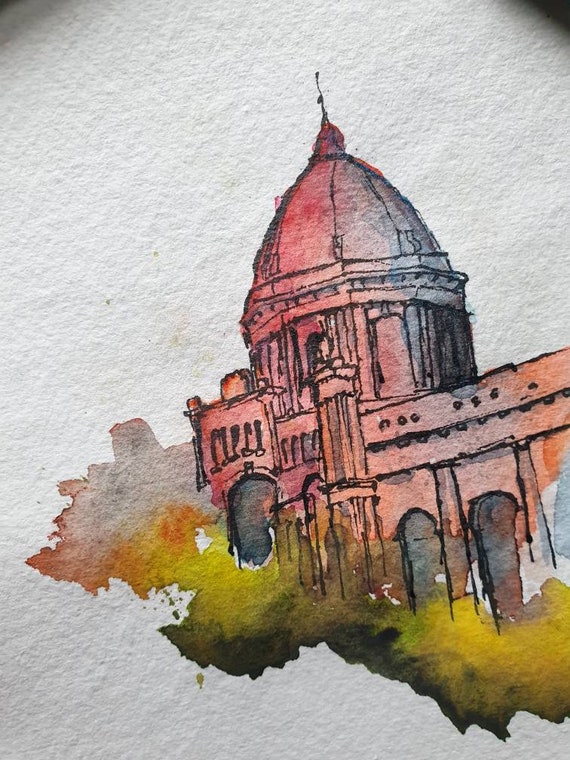This is a detailed watercolor painting of a grand building that closely resembles a U.S. Capitol building, characterized by its prominent domed roof, also described as a coppola or steeple, crowned with a point. The exterior of the building gradates from red to orange hues, creating a warm glow, particularly on the side illuminated by light, while the shadowed areas exhibit blue-purple tones. The structure features black ink outlines that define its intricate architectural elements, including multiple archways and oval openings. Some areas of the black outlines appear slightly smeared, enhancing the watercolor effect.

At the base of the building, there are organic, loosely defined foliage shapes that transition from green to yellow, which appear to blend into the shadows of the building itself. The painting rests on a piece of textured white watercolor paper, adding an additional layer of depth and authenticity to the artwork. The bottom part of the image features splashes of vibrant color, creating an almost ethereal, multicolored foundation that fades into parts of the building, enhancing the sense of motion and fluidity typical of watercolor paintings.